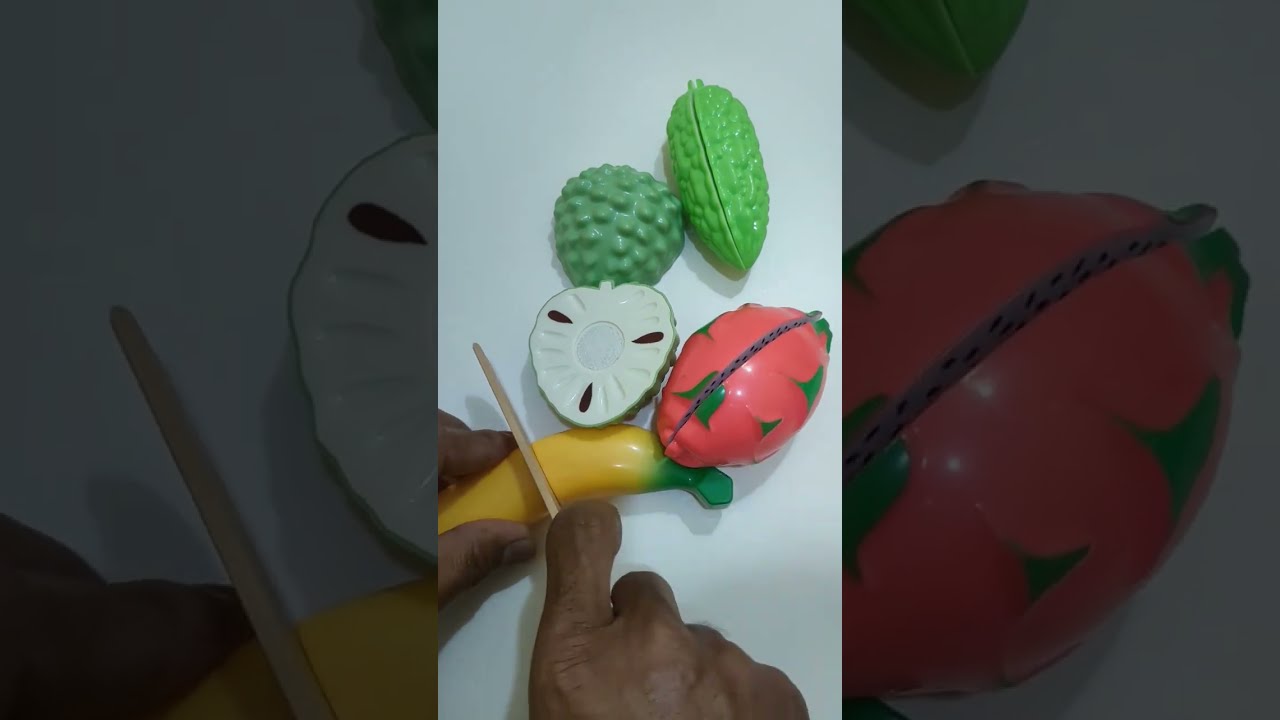In the image, set against a solid white background, we see an indoor scene that appears to be in a kitchen. The image is possibly a screenshot from a mobile device. Central to the image are various plastic fruits and vegetables, which are vividly detailed in colors such as green, yellow, tan, brown, and pink. Two hands are visible, with the right hand holding a brown plastic knife, poised to cut into a plastic yellow banana. The banana, marked by a seam down the middle, is being split using a wooden tongue depressor. Surrounding the banana is an array of other plastic fruits: a green pickle-like object with a seam, a green bumpy piece, a round pink and green fruit, a white strawberry-shaped fruit, and a nut-like object. All of these items rest on a white table, adding to the overall illusion of a real culinary scene. The meticulous details of the plastic seams and the placement of the fruit pieces create a playful, yet realistic depiction of a food preparation scenario.